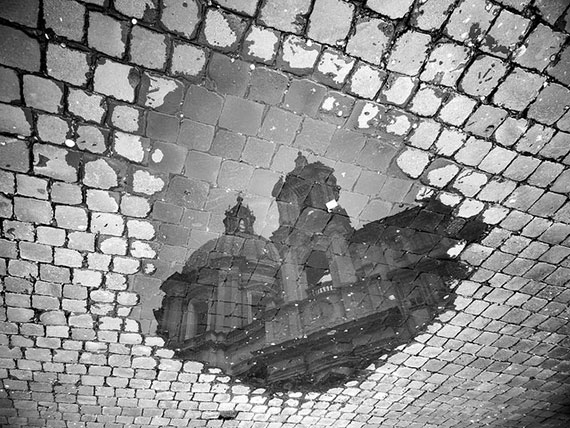This black and white photograph features a stone walkway composed of square tiles in a state of disrepair, with many tiles missing paint. Central to the image is a puddle that captures a detailed reflection of an architectural scene. The reflection reveals a grand palace or castle with large columns and a dome-shaped structure, possibly a church tower, adding a majestic feel to the scene. The artistry is so precise that it almost feels like a passage into a different dimension, providing a starkly clear and intricate nighttime view of this enchanting cityscape, complete with towering spires and official buildings. The overall composition, with its vivid and almost surreal quality, blends elements of both natural reflection and artistic rendering.